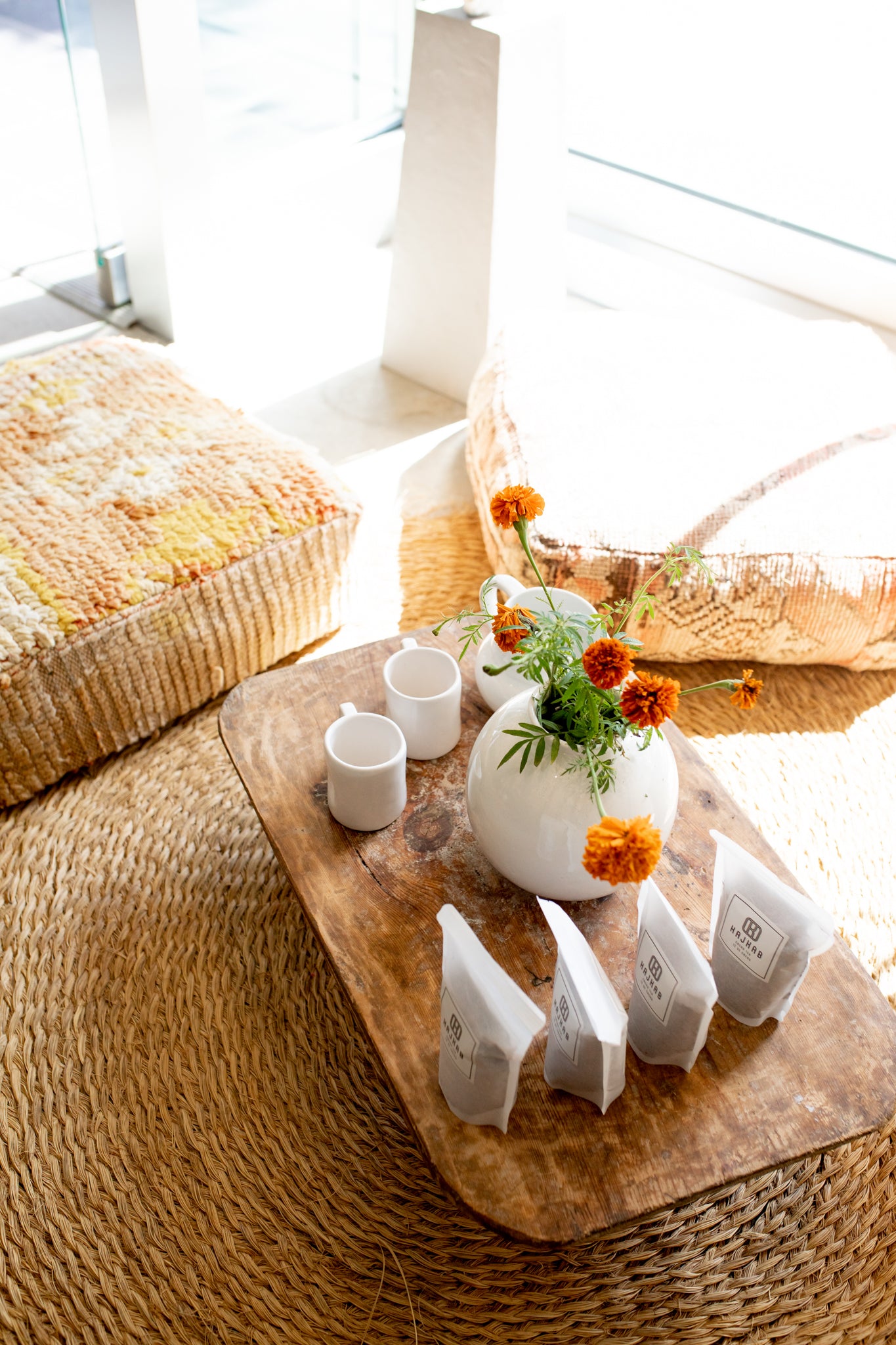This photograph captures a cozy living room setting bathed in natural daylight. At the center, a rustic wooden table hosts a beautifully arranged setup. On the left side of the table, a white teapot and two matching white mugs are positioned, untouched and awaiting use. The middle of the table is adorned with a white circular vase filled with vibrant orange marigolds, with one flower just beginning to bloom amid the others in full blossom. To the right, four upright packages—each labeled with what appears to be "H-A-J" or "N-A-J"—suggesting tea or coffee, align neatly. This wooden table is placed on a circular, woven burlap rug, enhancing the cozy ambiance. Earth-toned, fluffy pillows are scattered on the floor to the left and top quarter of the image, adding to the inviting atmosphere. The clear, natural light streaming in suggests it’s daytime, possibly illuminating the room through unseen glass windows, further contributing to the warm and welcoming mood.